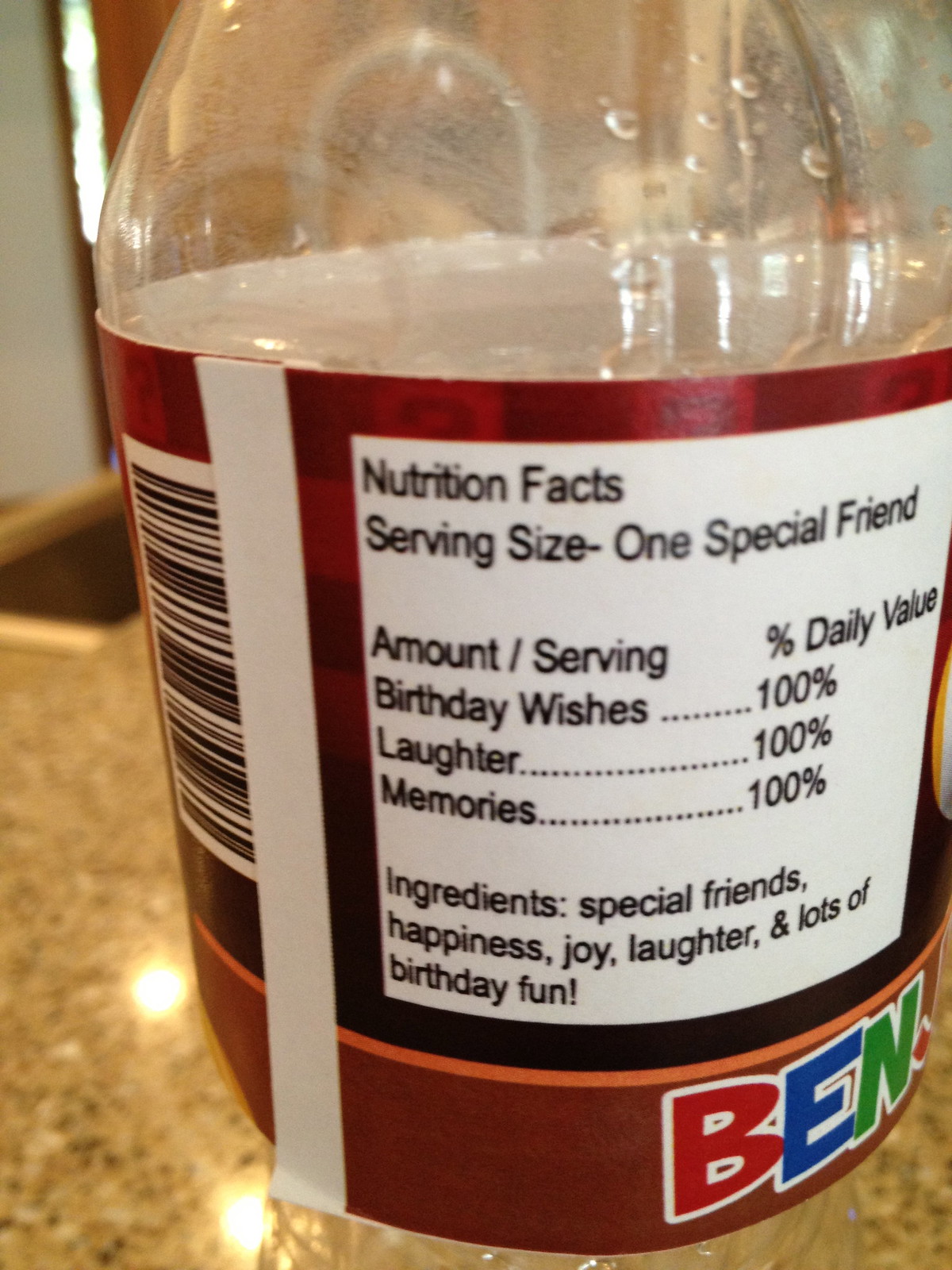This vertical close-up image features a plastic bottle on a dark brown countertop with black flecks, resembling granite. The bottle appears to be empty and has a label with detailed nutrition facts. The label's background is red and brown, with the name "BEN" prominently displayed at the bottom in colorful letters: the B in red, the E in blue, and the N in green, all outlined in white. The nutrition facts section lists a serving size of "one special friend" and includes whimsical values such as 100% for birthday wishes, laughter, and memories. Additionally, the ingredients listed are special friends, happiness, joy, laughter, and plenty of birthday fun. A barcode is visible on the side, and the bottle's top features clear plastic, allowing a peek inside.